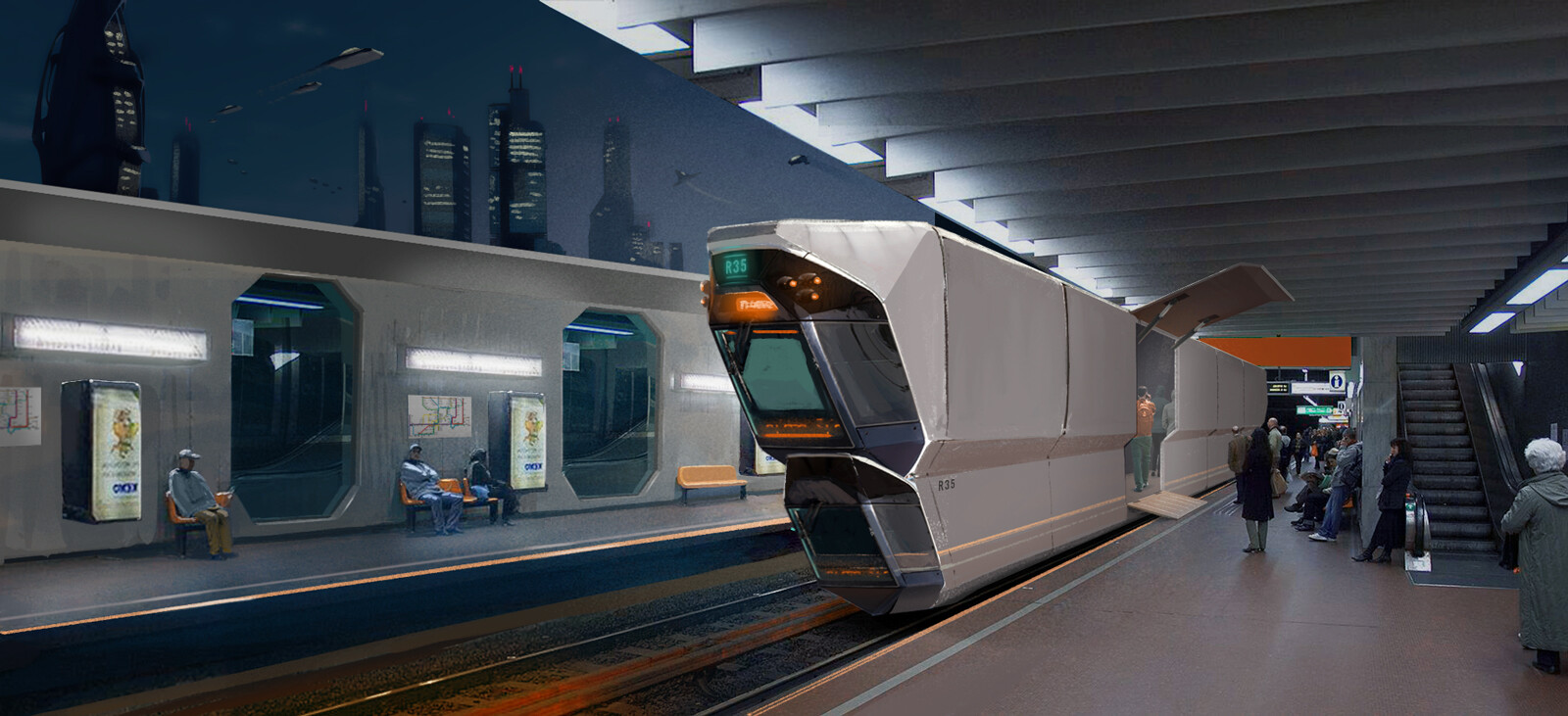The image captures the interior of a sleek, modern, and likely electric train station, possibly part of a futuristic public rail system. The scene is wide and horizontally rectangular. Dominated by dark blue walls with gray accents, the terminal is very spacious and has a contemporary feel. The center of the image features the sunken track area, designed for the train to glide along.

The centerpiece is a state-of-the-art train, crafted from gray metal with a distinctly angular design. The upper half of the train's front notably slants forward, creating a streamlined appearance. Black panels, featuring luminescent green and orange lights, adorn the front, along with small viewing screens. The train’s door is bifurcated; its top half lifts upward while the bottom half descends to the platform, facilitating passenger boarding. Several individuals are seen either entering the train or waiting nearby.

To the right, a sleek black escalator ascends, contributing to the station's modernist aesthetic. A bright white ceiling with numerous slats casts a soft light across the area. The floor is primarily gray, with sections appearing brown. On the left, a secondary waiting zone includes yellowish-orange benches and squared windows, set against a backdrop of towering dark structures and flying cars, reinforcing the futuristic atmosphere. Yellow fluorescent lights add a warm glow to the otherwise cool-colored environment, further emphasizing the high-tech, urban ambiance of the station.